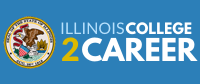The image is a detailed section of a website featuring a predominantly white background. Prominently displayed is a blue, horizontal rectangle. On the left side of this rectangle, there is a small, official-looking seal. While the exact details of the seal are difficult to discern, it appears to be the State Seal of Illinois, featuring an American Eagle holding a banner, a shield beneath the eagle, and a perimeter inscription which may indicate its state affiliation. The seal is outlined in yellow.

Next to the seal, the text "ILLINOIS COLLEGE TO KOREA" is displayed. The word "ILLINOIS" is written in light blue, non-bold, uppercase letters. Adjacent to it, "COLLEGE" appears in bold, white, uppercase letters, with no space separating it from "ILLINOIS." Beneath this, a large, yellow number "2" is prominently displayed, followed by the word "KOREA" in large, bold, white font. The overall layout combines these elements to focus viewers' attention on the "Illinois College to Korea" text, divided contextually by the seal and the numeral 2.